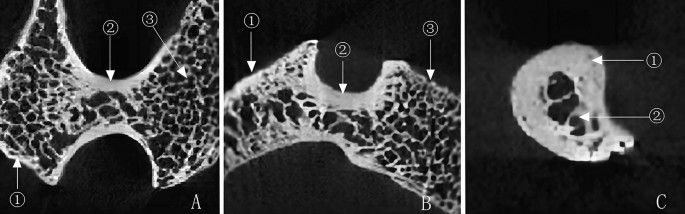The image display comprises three high-resolution grayscale x-ray images labeled A, B, and C against a completely black background. The x-rays appear to depict small, possibly curved bone fragments, characterized by visible porous structures and holes suggestive of spaces for bone marrow or collagen. Each x-ray is annotated with arrows pointing to specific areas of interest: images A and B each have three labeled points (1, 2, and 3), while image C has two (1 and 2). Image A features a butterfly-shaped bone, image B displays similarly annotated features, and image C showcases a bone fragment that is somewhat ear-shaped. The detailed close-up nature of these images makes it challenging to identify the specific bones or their locations in the body, but the annotations seem to highlight important morphological characteristics.